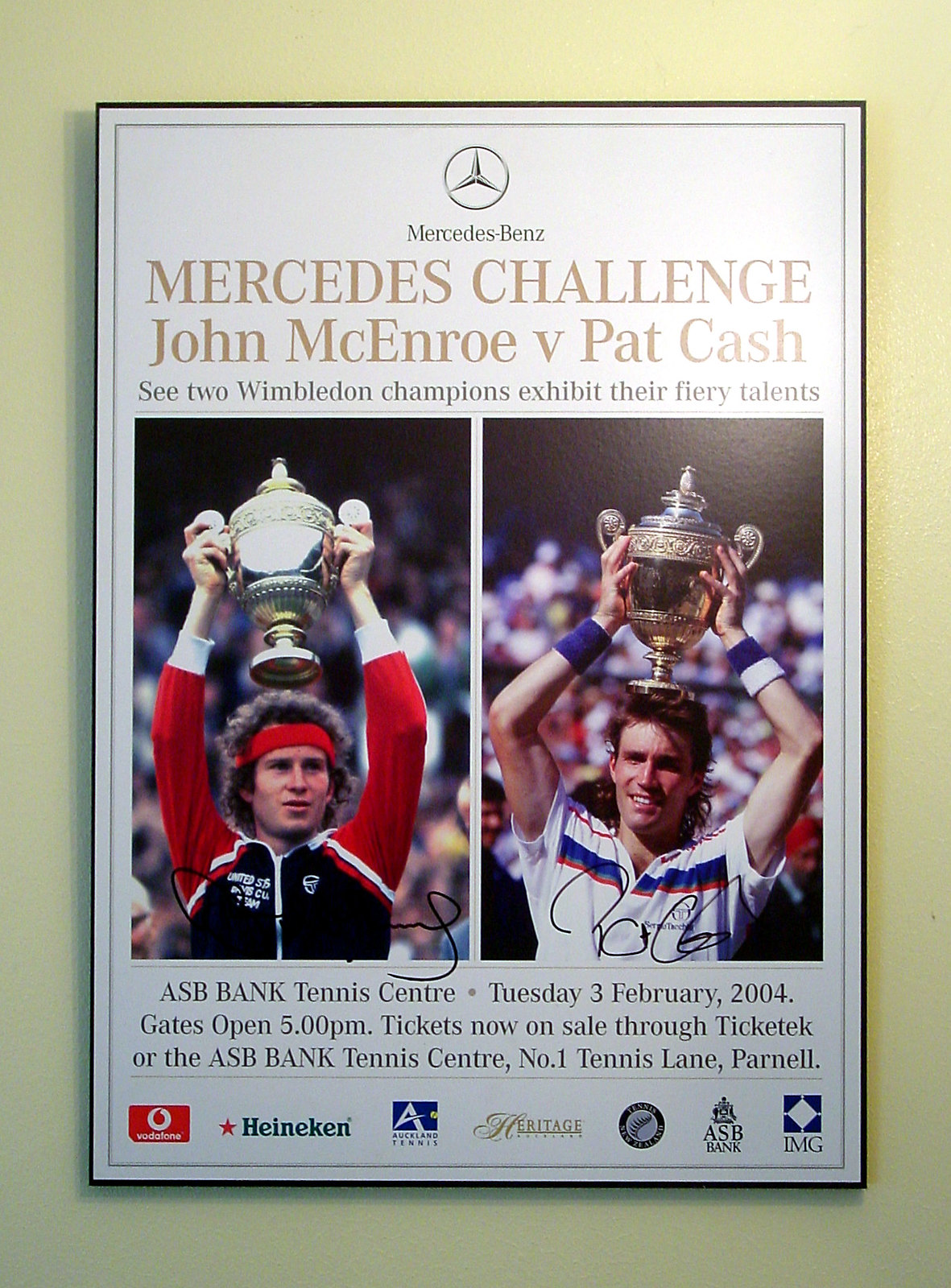The image is of a framed poster on a light yellow-beige wall, illuminated from the upper right. The poster is primarily white with tannish-brown text. At the top is the Mercedes-Benz logo and name, followed by the title "Mercedes Challenge: John McEnroe vs. Pat Cash." The tagline reads, "See two Wimbledon champions exhibit their fiery talents."

Below the text are two vertical photographs of John McEnroe and Pat Cash, each holding a large silver trophy overhead. John McEnroe, on the left, sports curly brown hair, a red headband, and a red and black tracksuit. Pat Cash, on the right, has long shaggy brown hair and wears a white shirt with blue stripes and blue wristbands. Both images appear to be autographed.

Further down, black text details the event specifics: "ASB Tennis Center, Tuesday, 3 February 2004, gates open at 5 p.m." and notes that tickets are on sale through Ticketek or the ASB Bank Tennis Center at number one Tennis Lane, Parnell. The bottom of the poster features various sponsor logos, including Vodafone, Heineken, Auckland Tennis, Heritage, ASB Bank, and IMG.